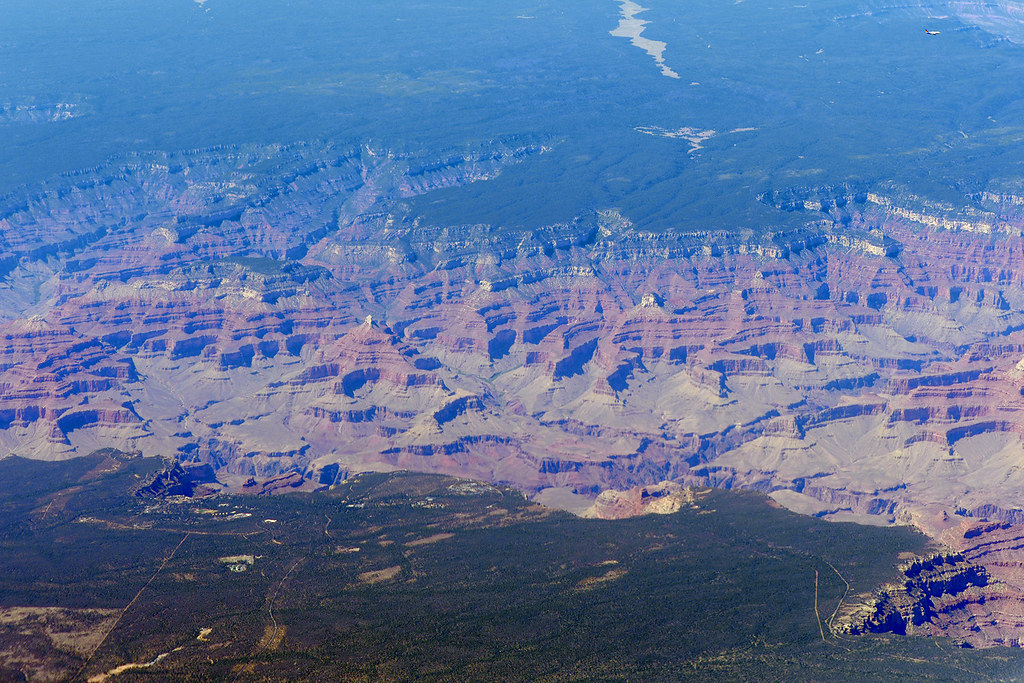This is a professional, high-altitude aerial photograph capturing a stunning landscape that might be the Grand Canyon. The image is likely taken from an airplane, a satellite, or possibly a high-flying drone. The extensive view showcases an expansive, reddish-brown canyon with steep, jagged cliffs that descend dramatically into the earth. Contrasting with the rugged terrain, the scene also features lush green areas filled with trees and vegetation. In the foreground, a flat green area abruptly falls away into the vast chasm below, creating a striking visual contrast. A winding, squiggly blue river meanders through the landscape, adding a splash of color. In the lower right-hand corner, a bright blue speck can be seen, although its exact nature is unclear. The photograph, devoid of any human or animal presence, captures the grandeur and isolation of this natural wonder. Additionally, a distant airplane is visible in the upper right-hand corner, suggesting the immense altitude from which this shot was taken. Overall, this image offers a detailed and breathtaking glimpse into the raw beauty of a monumental canyon landscape during daylight hours.